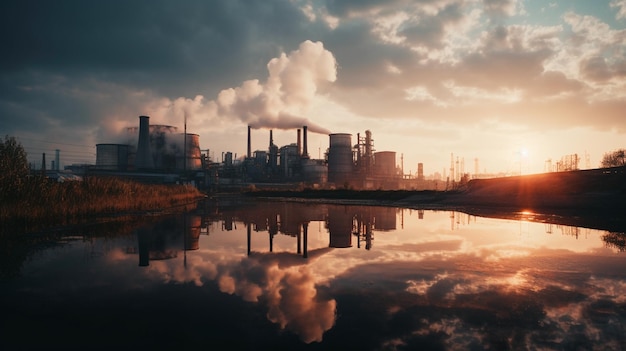This AI-generated image features a serene body of water in the foreground, perfectly mirroring an extensive industrial compound situated at the water's edge. The industrial area, which could be an oil refinery or smelting plant, includes large cylindrical buildings and reserved tanks, particularly noticeable on the left side. Billowing white smoke from multiple smokestacks adds an active dimension to the scene. The photo, taken horizontally, captures a stunning sky where the setting or rising sun creates a warm orange glow that gradients into various shades of blue. The golden, blue, gray, and white clouds further enrich the sky's texture, enhancing the overall ambiance. Despite its industrial nature, the scene has an almost surreal quality due to the unnaturally smooth and still water, reflecting the entire landscape like a polished mirror. A small grassy plain occupies the left-hand side of the frame, adding a touch of nature to the industrial backdrop.